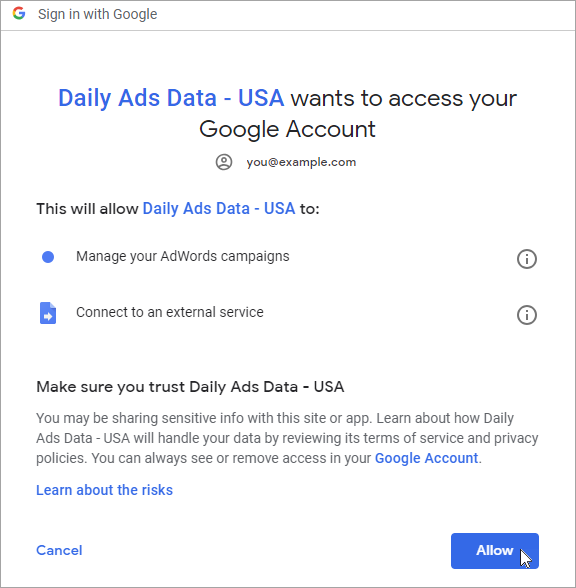The image depicts a Google sign-in request interface for an external service. The interface features a white box with a black border. At the top, the text "Sign in with Google" is prominently displayed. Below this, the service "Daily Ad Data USA" is mentioned in blue text, indicating that it wishes to access the user's Google account.

The central message, in black text, states: "Daily Ad Data USA wants to access your Google account." It specifies that by signing in, the service will be able to manage the user's AdWords campaign and connect to an external service, each followed by an information icon represented by a circle containing a lowercase "i."

Further down, there is a prompt in black text advising users to ensure they have chosen "Daily Ad Data USA." Another line cautions that sharing sensitive information with the site or app is possible. Users are encouraged to review the service's terms and privacy policies to understand how their data will be handled. A reminder follows that users can always view or revoke access in their Google account, with "Google account" being a blue hyperlink.

Below this reminder, additional blue hyperlinks with the text "Learn about the risks" and "Cancel" provide options for further information or to cancel the permission request, respectively. At the bottom, a central button with a blue background is labeled "Allow," indicating the action to grant the requested permissions.